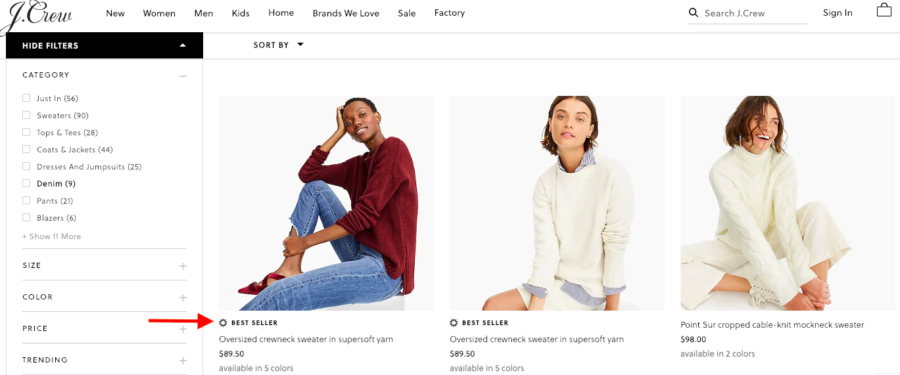Screenshot of the J.Crew homepage featuring a clean, pure white background. Centrally positioned is a "Bestseller" section showcasing three male models. The first model on the far left is wearing a red sweater, blue jeans, and red socks, with a red arrow pointing to him indicating a bestseller item. The second model, in the middle, sports a white sweater layered over a blue undershirt, paired with khakis—a combination also tagged as a bestseller. The third model, on the right, is wearing an outfit similar to the second model, further emphasizing the popularity of the look. At the top of the page, you can see options to 'Search', 'Sign In', and several filters for sorting by size, color, price, and trending items. This section is designed to help users quickly navigate to desired categories, particularly within menswear.